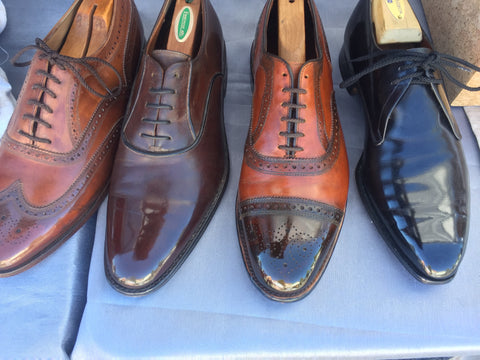The image is a top-down shot of four pairs of men's dress shoes arranged adjacently on a silvery blue-colored background. Each pair features wooden shoe trees. From left to right, the first pair is a typical English tan leather brogue with a weathered look and brown laces, exuding a shiny finish. The second pair is a dark brown oxford with horizontally laced strings and a striking high-shine on the tip of the toe, accompanied by a shoe tree with a green label. The third pair is a two-toned brogue with a darker tip and round laces, showcasing a unique blend of colors. The final pair is a sleek black oxford, extremely shiny, possibly patent leather. The image is visually appealing with a muted pastel tone, suggesting it was taken under diffused, possibly outdoor lighting. The luxurious appearance of the shoes and the meticulous arrangement hint at their high value and classic style.